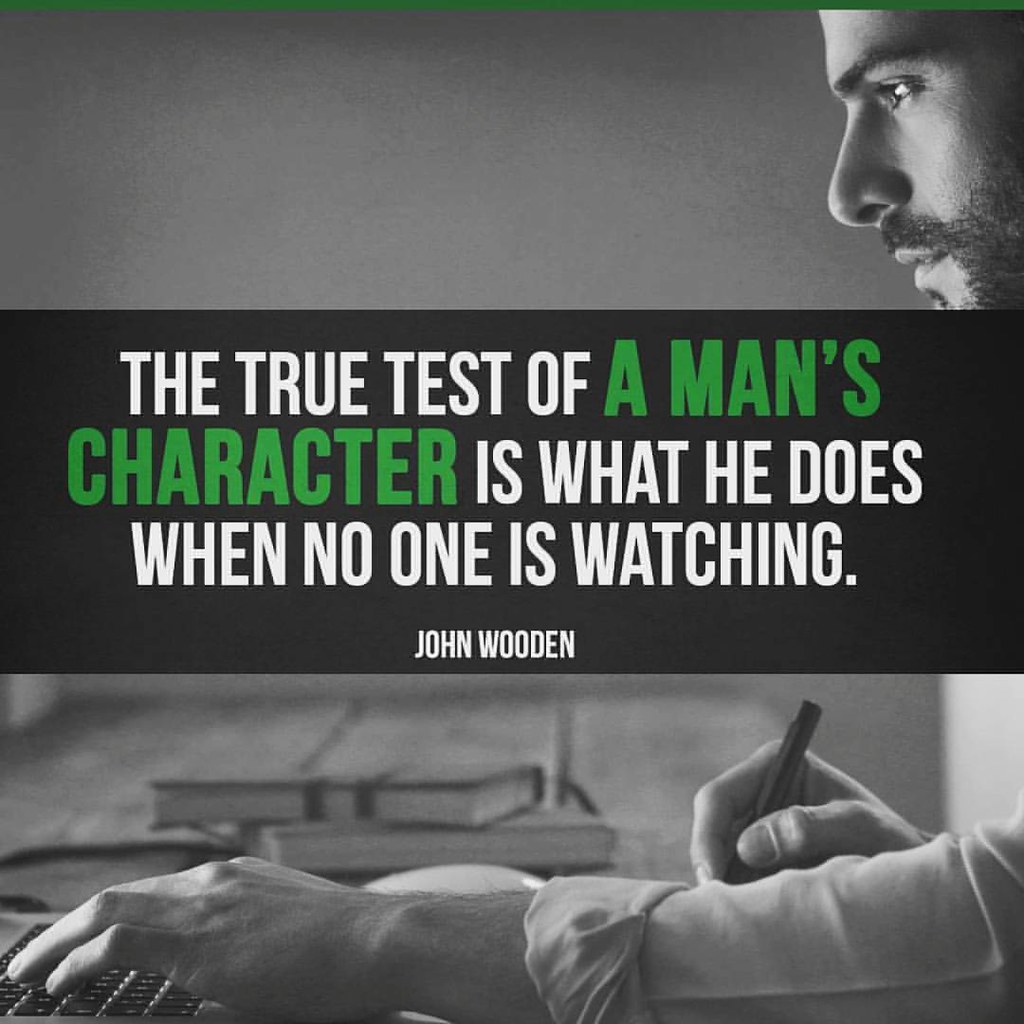The black and white image showcases a man seated at a desk, focusing on his work. His face is positioned in the top right corner of the image, captured from a side profile, highlighting his beard and concentrated expression. With one hand, he types on a laptop keyboard, while the other hand holds a pen, indicating he is multitasking or deeply engaged in his work. Leather-bound notebooks are neatly placed on the desk beside him, adding to the scholarly atmosphere. Dominating the center of the image is a black banner with a motivational quote that reads, "The true test of a man's character is what he does when no one is watching," attributed to John Wooden. The white and green text on the banner contrasts strikingly with the monochrome background, making it stand out. This square photo resembles graphics often shared on social media platforms, designed to inspire viewers with an uplifting message.